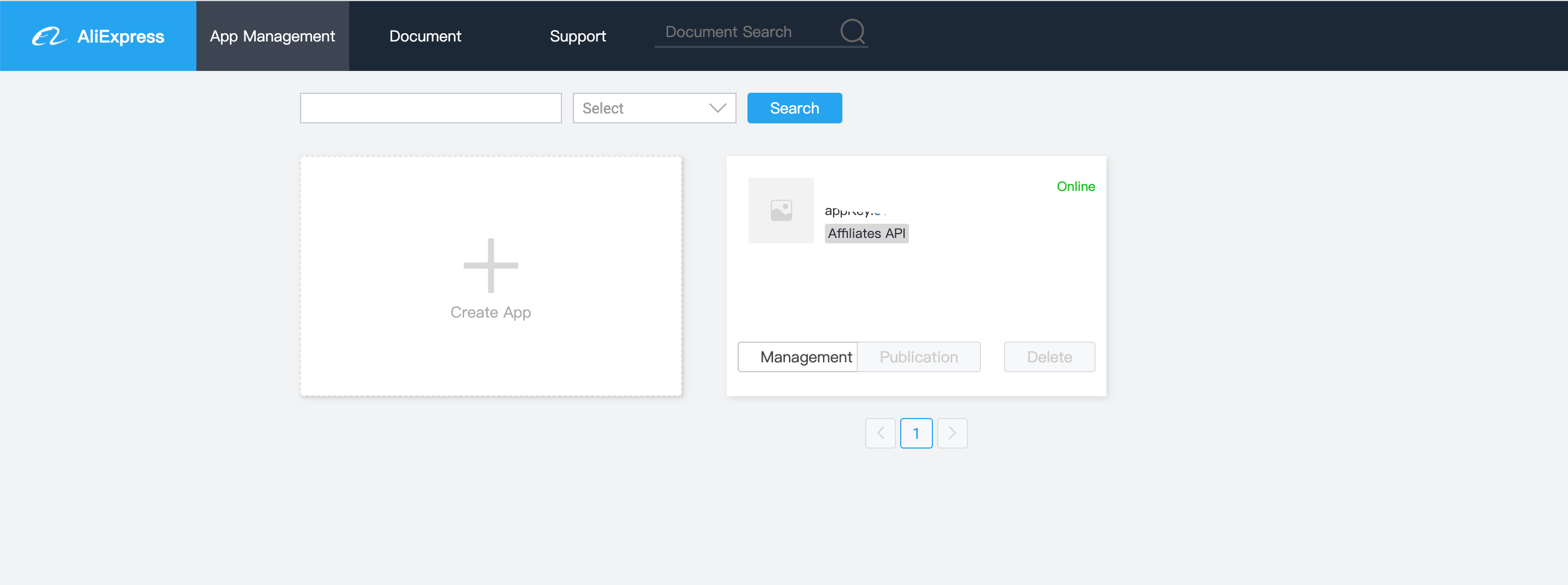The image showcases an interface of an app management software. At the top, set against a black taskbar, the far left section is highlighted in blue with "AliExpress" written in white font. To its right, within the darker segment, the text "App Management” is visible, followed by "Document," and "Support." 

Prominently placed beneath this bar is a white search area that includes a search bar labeled "Document Search." Below it, occupying the lighter section of the screen, is an empty text box. Adjacent to this is a drop-down menu titled "Select," and beside it is a blue tab labeled "Search."

Further down, the interface displays a larger rectangular box featuring a plus sign and the text "Create App.” Next to it is another box with the phrase "Affiliate API," detailing functions at the bottom such as "Management," "Publication," and "Delete." At the very bottom of the interface, it is marked with a "One,” possibly indicating the current page number within the application.